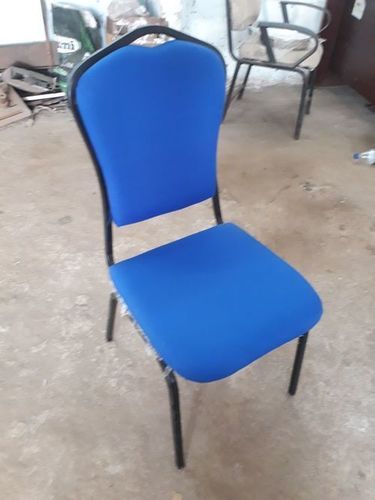The image features a prominently-placed bright blue chair with black legs and a black diamond-shaped frame at the upper back, situated in the center and facing east on a gray, smudged cement floor. Additionally, there is a gray chair with similar black components, located in the top right corner of the image, positioned towards a dark brown door. The background, particularly the top left corner, contains a mixture of clutter including a gray rectangular tray, a sand tray, and a dark green paper bag. Further back, there are hints of wooden debris and possibly a cardboard box. A water bottle with a blue cap is visible on the right-hand side of the image. The setting appears to be indoors, potentially a home or office, and the overall state of the floor and the scattered items suggest a rather disorganized environment.